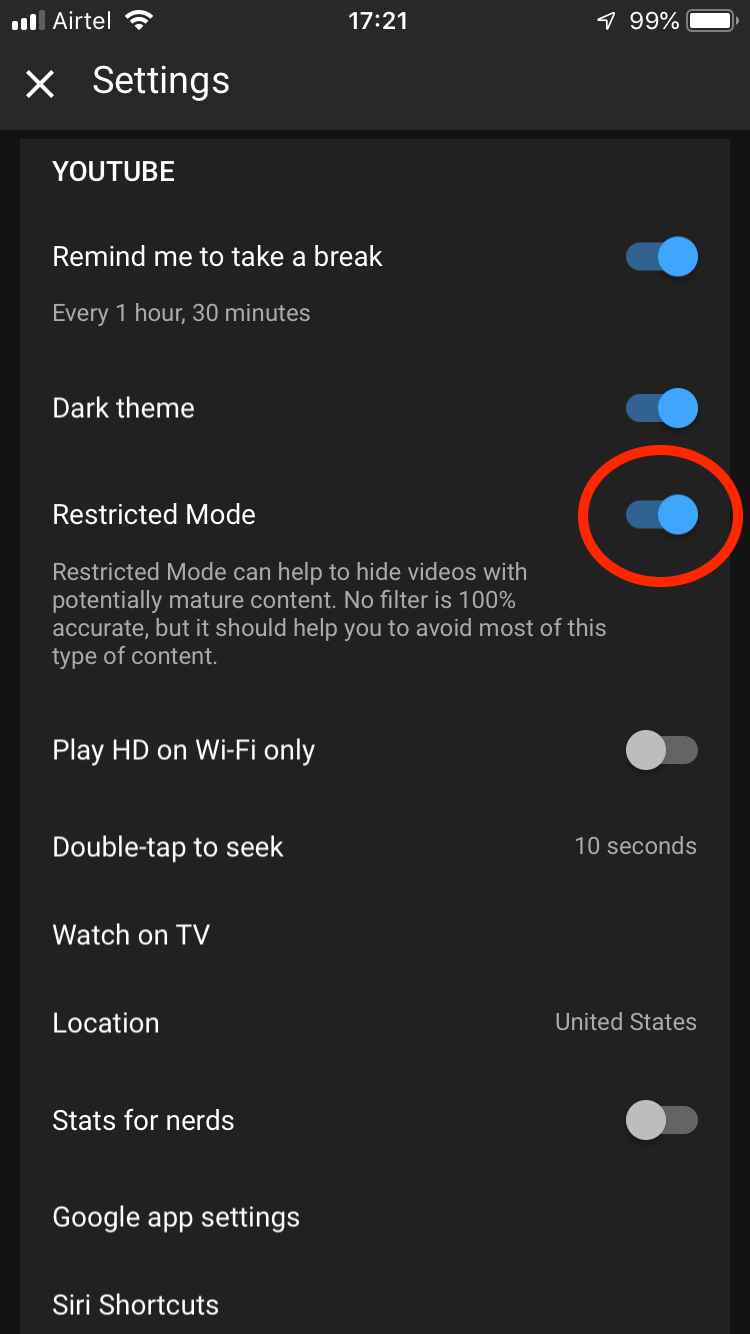This detailed image depicts a screenshot of the YouTube settings menu. At the top, there is a "Settings" label with a white "X" icon to the left, allowing users to exit the menu. Directly below this, we see a section titled "YouTube."

In this section, several settings are listed:

1. **Remind me to take a break**: This feature is enabled and set to remind the user to take a break every 1 hour and 30 minutes.
2. **Dark theme**: This setting is also activated.
3. **Restricted mode**: Enabled as well. This particular setting is highlighted with a red circle around the blue toggle, indicating it is on. A description beneath this option explains that Restricted mode can help to hide videos with potentially mature content. Although no filter is 100% accurate, it should help to avoid most mature content.

Further down the menu, the following settings are visible:
- **Play HD on Wi-Fi only**: This option is turned off.
- **Double tap to seek**: Set to 10 seconds for easier video navigation.
- **Watch on TV**: This does not appear to be toggled or changed.
- **Location**: Set to the United States.
- **Stats for nerds**: This feature is turned off.
- **Google app settings** and **Siri shortcuts**: These options are listed at the bottom of the screen.

The time displayed at the top of the screenshot is 17:21, and the phone's battery is nearly full at 99%.